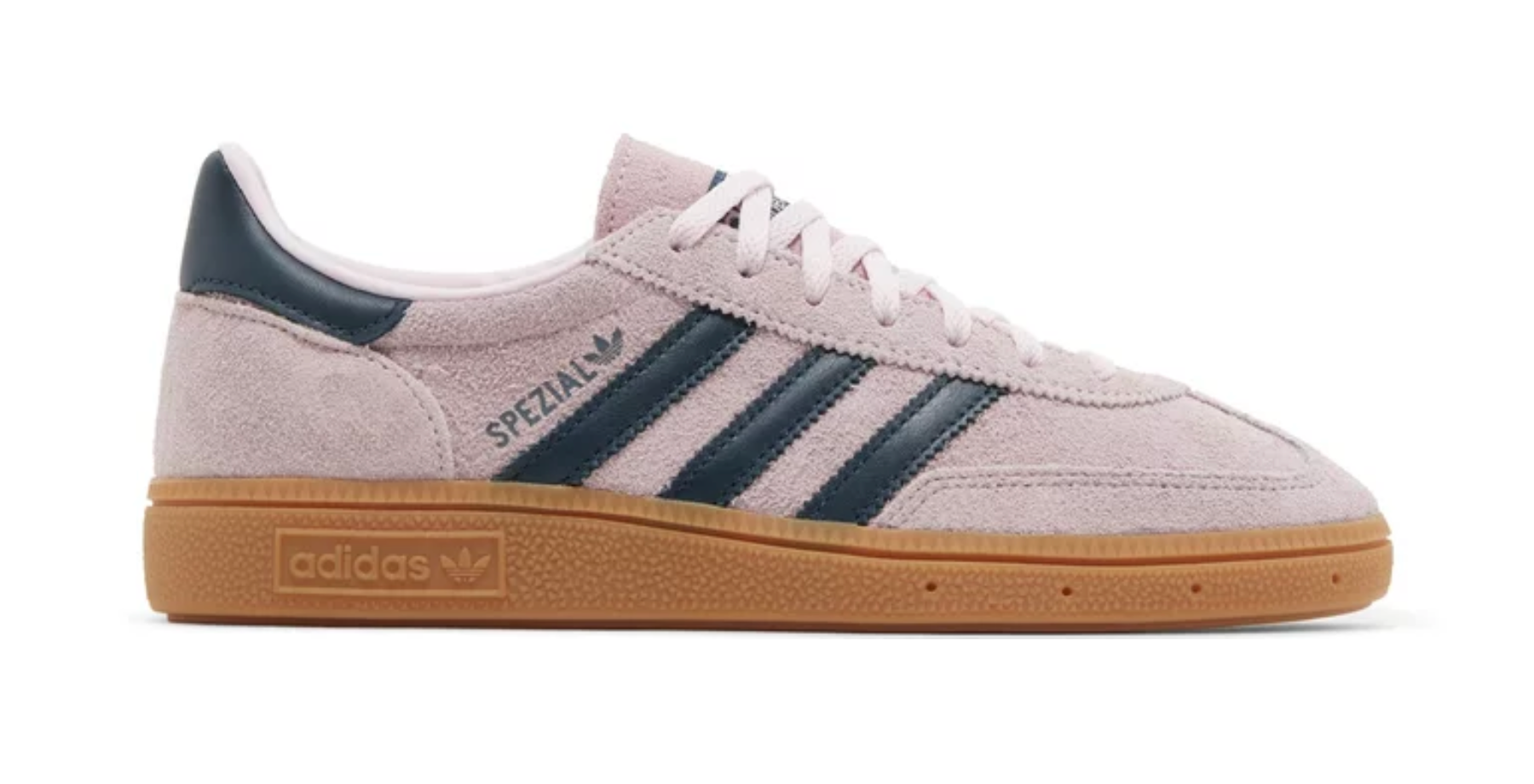This photograph showcases a single Adidas sneaker set against a pristine white background, giving it a floating appearance. The sneaker is oriented from left to right, revealing its predominantly off-white body accentuated by three distinct diagonal black stripes on the side. These stripes are complemented by the word "SPEZIAL," positioned just behind them, flanked by the classic Adidas logo.

The sneaker features a robust brown sole, detailed with an imprint of the Adidas brand name along with the company's iconic three-leaf graphic. Notably, the heel area is adorned with a black band, contrasting with the shoe's otherwise neutral color palette. The sneaker boasts crisp white laces and a comparatively brighter inner lining that peeks through, providing a subtle contrast to its exterior.

Overall, the clean, minimalist background emphasizes the design and craftsmanship of the sneaker, highlighting every intricate detail from the textured sole to the branded elements.